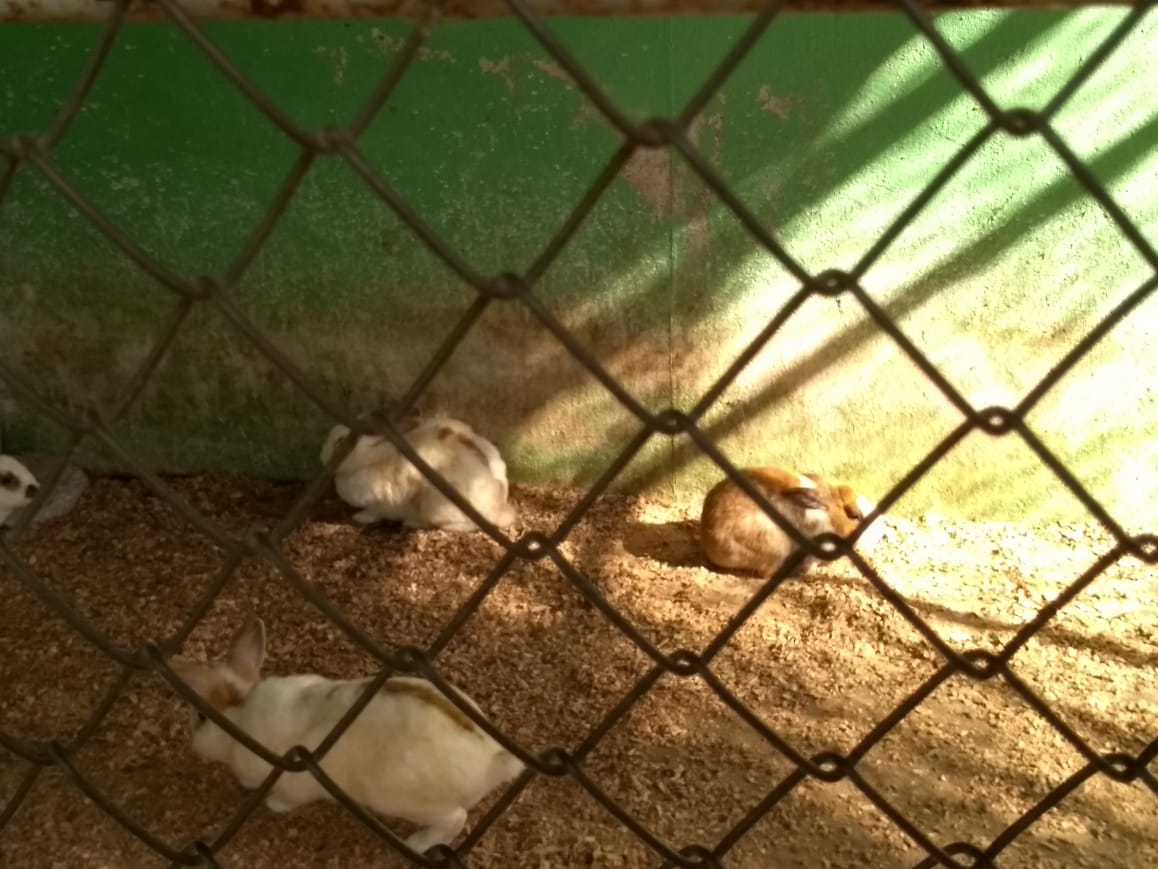The photograph captures an outdoor scene viewed through a chain-link fence, partially obstructing the image. Behind the metal fence, a trio of bunny rabbits can be seen on a light brown, sandy, and rocky surface. Two of the rabbits, larger in size and predominantly white with brown markings, are positioned towards the left. One of these rabbits appears to be running away towards the left edge of the photograph, while the other is near the green wall in the back. This wall, badly peeling with remnants of chipped paint revealing patches of yellow, brown, and white, forms the background of the image. The sunlight streaming in from the upper right casts diagonal shadows of the fence onto the weathered wall. Another rabbit, light brown in color with darker brown ears, is situated more towards the right section of the image, appearing hunched over. Barely visible, a fourth rabbit with brown markings around its eyes peeks from the far left. The ground is a mix of compact dirt and scattered rocks, illuminated by the sunlight filtering through the fence.